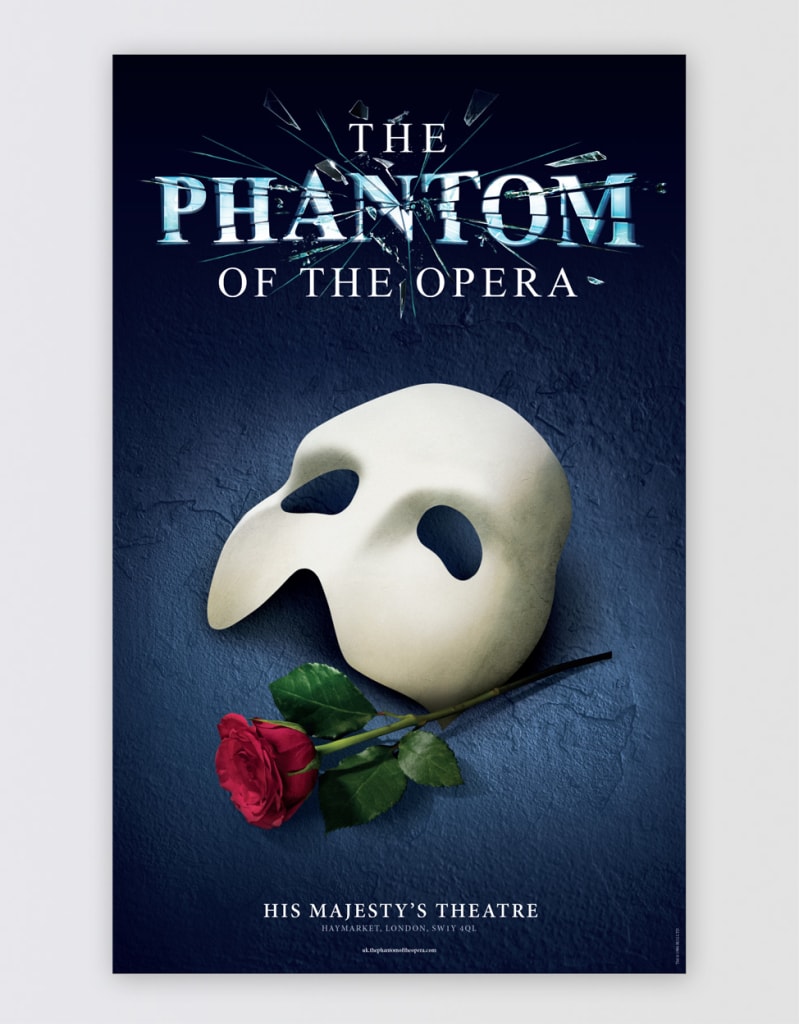The poster for "The Phantom of the Opera" is strikingly centered on a blue textured background. At the top, the title "The Phantom of the Opera" is prominently displayed in white text, with the word "phantom" featuring a shattered glass dual-tone effect in white and blue. Dominating the center is the iconic white phantom mask above a red rose tilted at a 45-degree angle, complete with a green stem and leaves. Below the rose, in smaller white text, it reads "His Majesty's Theatre, Haymarket London, SW1Y 4QL." Additional text, possibly a website or further details, appears in even smaller print below this line but is not legible. The poster is framed with a subtle vignette effect at the top and bottom, keeping all elements impeccably aligned and centrally focused.